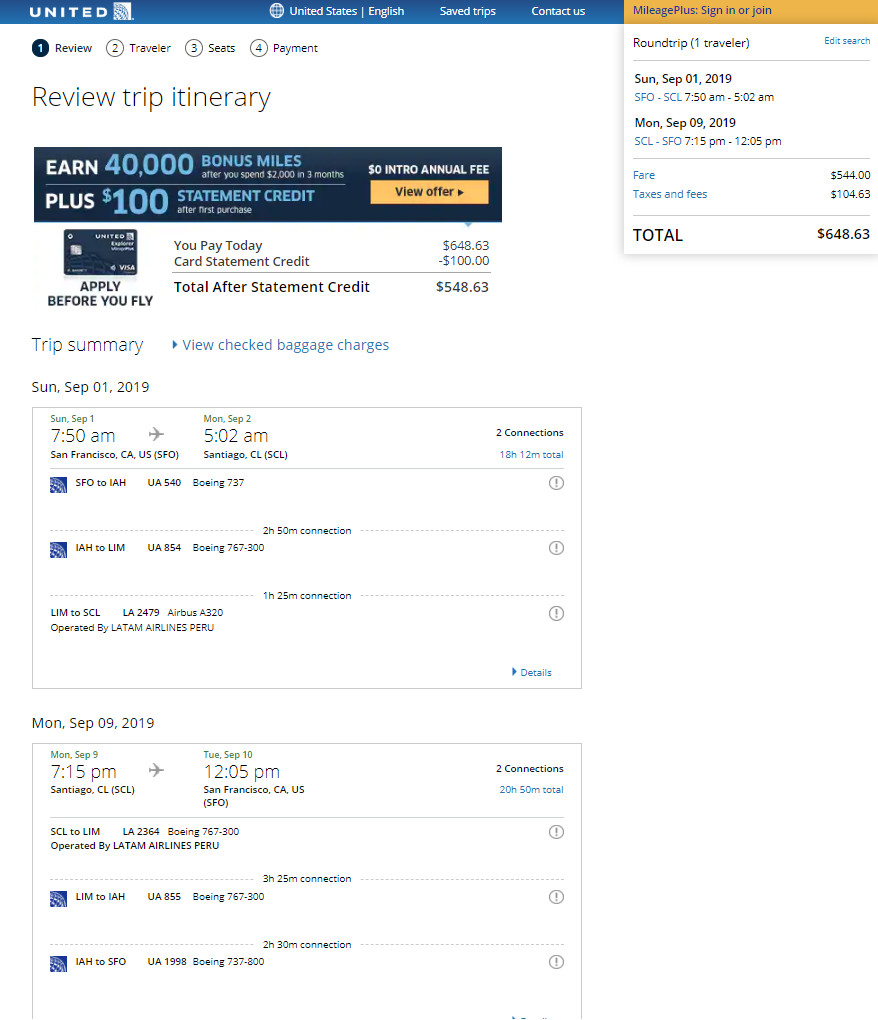This is a detailed screenshot of a website for United Airlines. At the very top, there's a blue navigation bar featuring the text "United" in white font, followed by "United States - English" next to a white globe icon. On the same bar, options for "Save Trips" and "Contact Us" are also displayed.

Beneath the navigation bar, in black font on a white background, the header reads "Review Trip Itinerary." 

Below this header, there's an advertisement for a credit card presented within a navy-blue rectangle. The advertisement prominently highlights in white font "Earn," followed by "40,000 Bonus Miles" in blue font. Additionally, it mentions a "0% Intro Annual Fee" in white font. 

Positioned below the main advertisement text is a yellow rectangular button that says "View Offer" in black font. Underneath the button, the text elaborates further in white font with "Plus" and then in blue font, "$100 Statement Credit after the First Purchase."

Accompanying the advertisement is a smaller image of a blue credit card adorned with the "United" logo. The financial summary indicates "You Pay Today: $648.63," then shows "Card Statement Credit: -$100," culminating in a "Total After Statement Credit: $548.63."